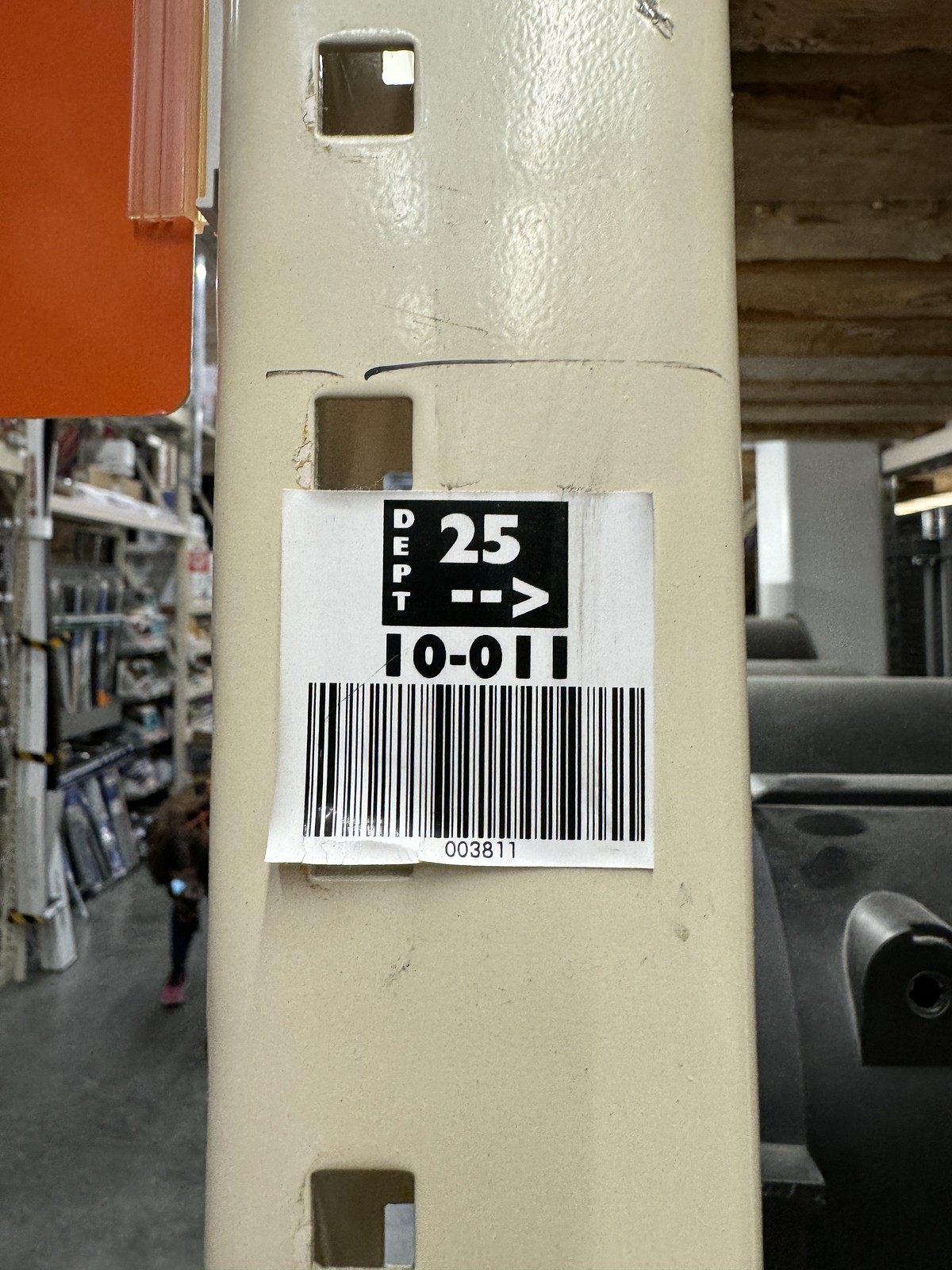This image captures the interior of a warehouse, prominently featuring a light tan structural pole in the center. Affixed to the pole is a white sign with a black square, displaying "DEPT 25" in white letters, accompanied by a dotted arrow pointing to the right. Below this, the sign reads "10-011" and includes a barcode. Adjacent to the sign, a plastic holder with an orange placard is attached to the pole's left side, with the placard's text facing away from the camera. In the background, shelves lined with pegboards hold various items. Partially obscured by the pole, an individual's leg is visible as they walk by, contributing to the bustling atmosphere of the warehouse.